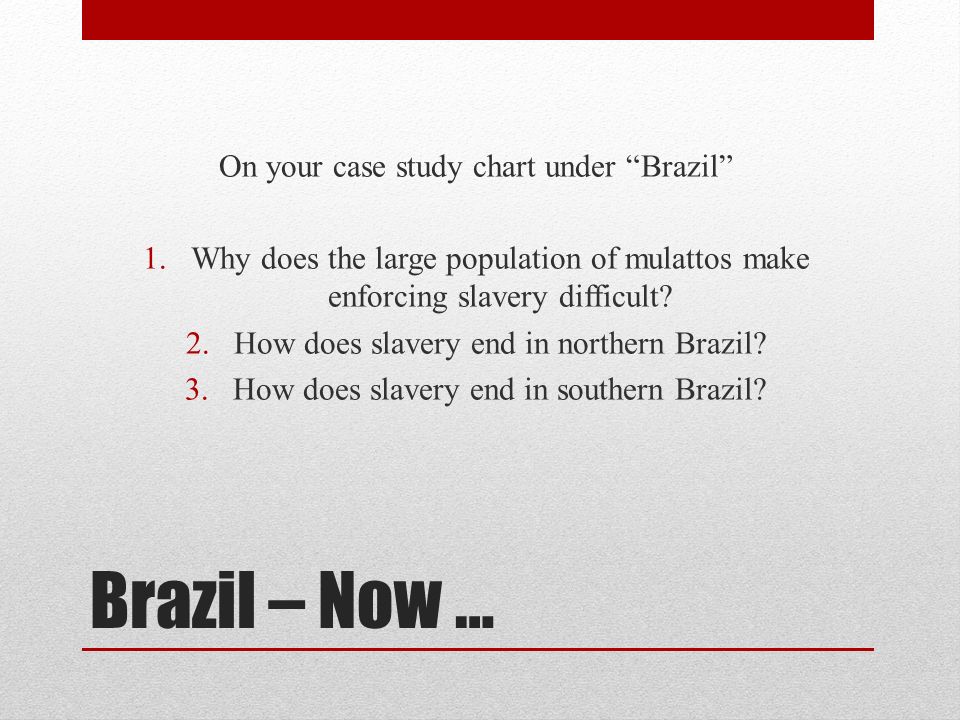Centered at the top of the page, a bold red bar stretches horizontally, flanked by white margins on either side. Below this, the background transitions to a very light gray, creating a subtle contrast. Prominently displayed in black letters, the heading reads, "On Your Case Study Chart - Brazil." Underneath, in numbered red text, there are three study prompts:

1. "Why does a large population of mulattoes make enforcing slavery difficult?"
2. "How does slavery end in Northern Brazil?"
3. "How does slavery end in Southern Brazil?"

A significant blank space follows these questions, leading to another bold heading in black text, "Brazil - Now..." Below this heading, a thin red line runs across the page. The remainder of the page is left intentionally blank, seemingly reserved for note-taking or responses. The overall color scheme of the page is dominated by red, white, gray, and black, indicating a study or review format aimed at understanding aspects of Brazilian history related to slavery.